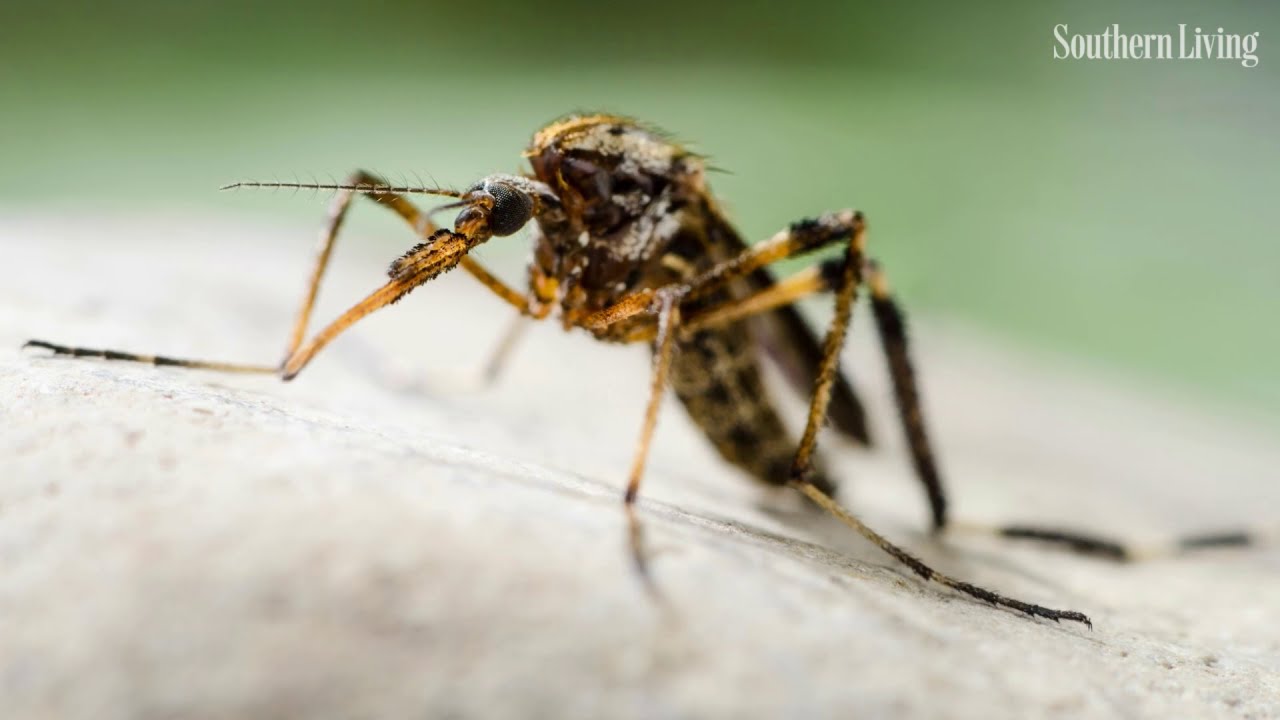This photorealistic image captures a highly detailed, close-up view of an insect, potentially a wasp, termite, or mosquito, with its striking features prominently displayed. The insect, centered and slightly turned three-quarters to the left, has a long, raised body adorned with a mix of gold, brown, and black hues. It boasts large, prominent black eyes and a distinct hump-like shape on its torso. The insect's six tall legs, three on each side, are bent in the middle and are vividly striped in gold and black. The insect's back tapers with lower wings visible, adding to its detailed anatomy.

The surface below is out of focus and light-colored, resembling sand, while the blurred, diffused background is a solid green, ensuring that the insect remains the focal point. The entire photograph exudes a magazine-like quality, heightened by the partially transparent white text "Southern Living" positioned in the top right corner against the green blur. The extreme close-up nature of the photo results in a slight loss of finer details but beautifully emphasizes the insect's striking and vivid features against an almost abstract background.